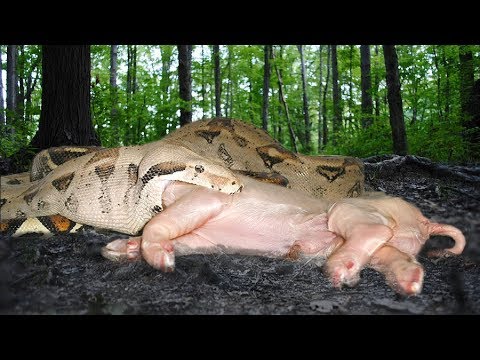This detailed photograph captures a Burmese python in the midst of devouring a young pig within a forest setting, possibly a wildlife refuge, zoo, or sanctuary. The forest floor, rugged with dark gray and black rocks, adds to the wild ambiance with its dirt and greenery. The python, with its tan and dark brown splotched body, has detached its lower jaw to envelop the medium-sized, lifeless pig, whose head and shoulders have already been consumed. Both animals are surrounded by a dense backdrop of green trees and glimpses of light peeking through, further emphasizing the naturalistic setting. The python's substantial length is apparent as it coils its long body in the background, underscoring its impressive size and the feat of consuming an animal larger than itself.